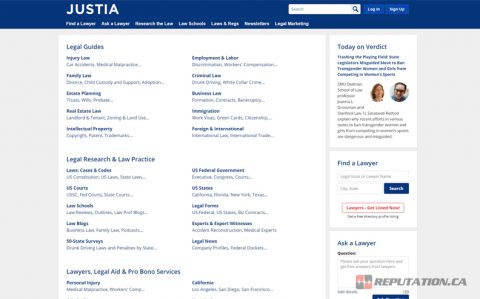This screenshot from the Justia website (www.justia.com) displays a comprehensive legal resource hub with a well-organized layout. At the top, a blue rectangle features clickable areas for navigation. As you scroll down, the central section highlights various legal categories, including "Injury Law," "Family Law," "Estate Planning," "Real Estate Law," "Intellectual Property," "Employment and Labor," "Criminal Law," "Business Law," "Immigration," and "Foreign & International Law." Additional sections offer "Legal Research" and "Law Practice" resources. Users can explore "Law Cases and Codes," "Courts," "Law Blogs," and "Learn About the Law." There's practical information like "Legal Aid and Pro Bono Services." The site also features current legal opinions in "Today on Verdict" and includes options to "Find a Lawyer" and "Ask a Lawyer," ensuring a broad spectrum of legal assistance and information is readily accessible.